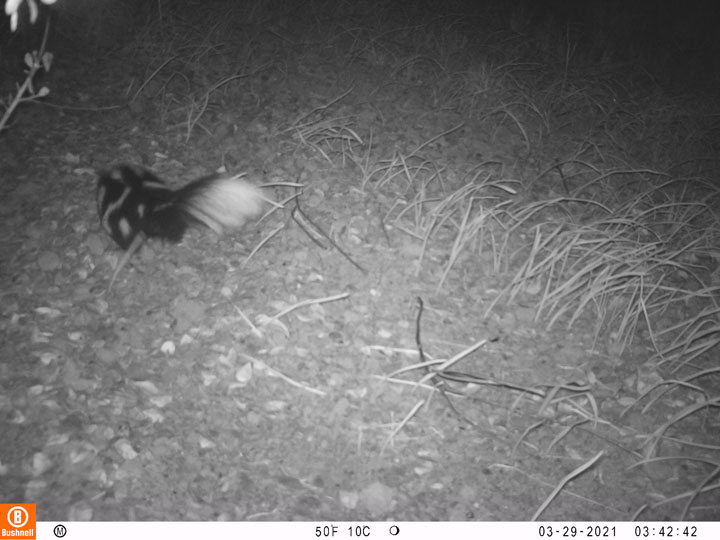The black and white photograph, likely captured by a night vision security camera, shows a skunk or a similar animal, such as a badger, walking away from the camera. The skunk is identifiable by its black fur with distinctive white stripes and a prominent white-tipped tail. The scene takes place in a field with dry grass and scattered leaves or petals on the ground that the skunk appears to have traversed. At the bottom of the image, there's an orange square featuring a white circle with a 'B' inside, labeled "Bushnell." Additional information displayed includes the temperature readings of 50 degrees Fahrenheit and 10 degrees Celsius, along with a date and time stamp: March 29, 2021, at 03:42:42.